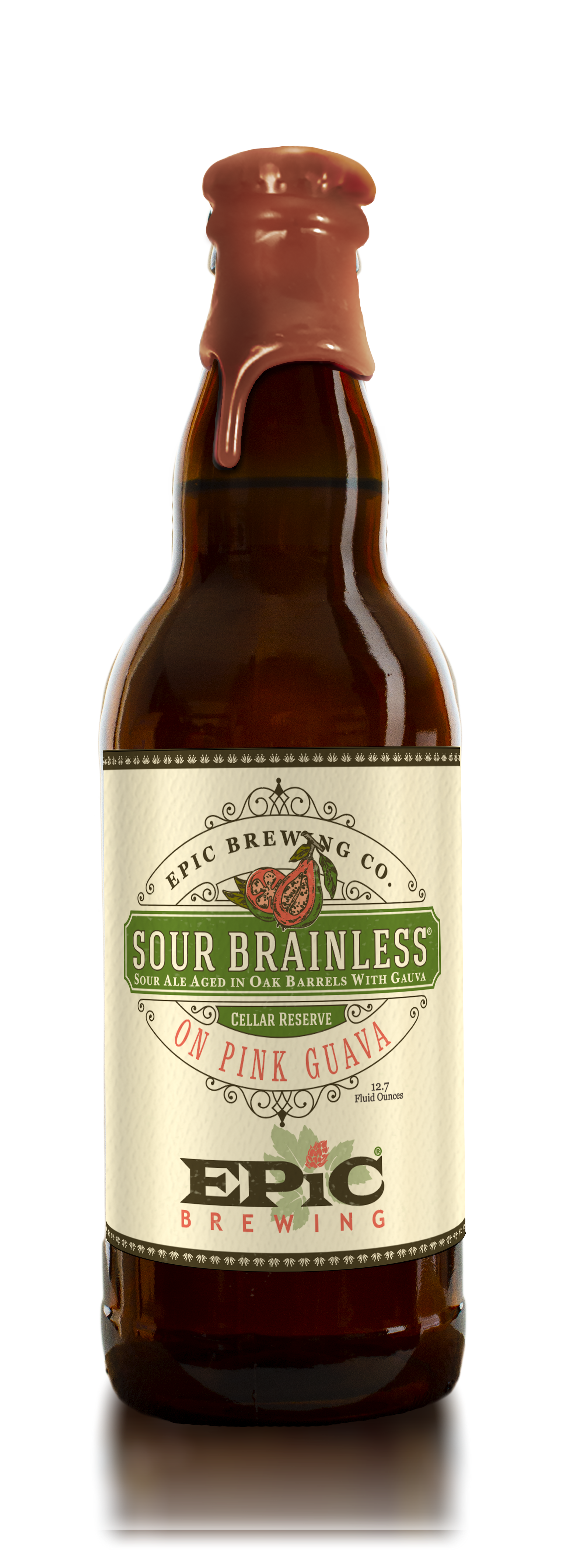This photograph captures a brown beer bottle with a distinctive red-brown hue and an intricate seal reminiscent of melted wax, similar to Maker's Mark, that extends about an inch and a half down the neck of the bottle. The label on the bottle is cream-colored with an olive green perimeter, adorned with detailed text and logos. At the top of the label in white letters on a green background, it reads "Epic Brewing Co." Below that, the main feature text announces the beer as "Sour Brainless" with the description "Sour ale aged in oak barrels with guava." Additionally, it notes "Cellar reserve on pink guava" in pink letters. The bottle’s capacity is listed as 12.7 fluid ounces. The carefully branded label also features some contrasting red and brown tones and includes the “Epic Brewing” name prominently in big black and red letters, making it a distinctive and eye-catching bottle.